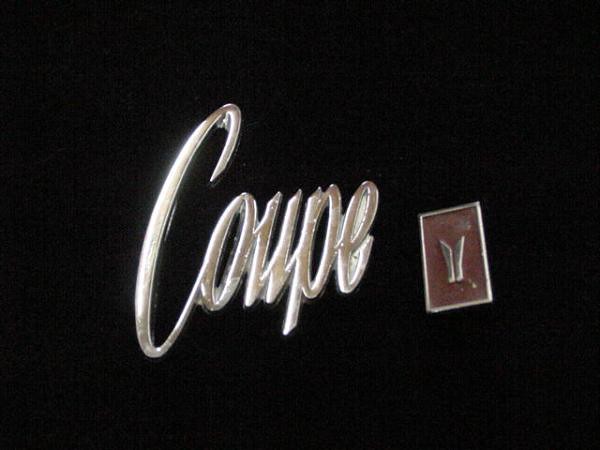The image features a completely black background, which could be either a piece of paper, cloth, or even the surface of a car. Centered prominently is an emblem with the word "COUPE" spelled out in capital letters. The word is designed to appear almost metallic, with a shiny gold-like finish, though it might be synthetic. The letters "C-O-U-P-E" are written in a cursive or elegant font, suggesting a refined or luxurious feel.

Adjacent to this central emblem is another smaller rectangular emblem. This rectangle has a silver border, enclosing a brown or red background that appears slightly dirty or worn, hinting at some age or weathering. In the center of this rectangle is a distinctive, symmetrical wing-like design, which gives an impression of motion or prestige. The two emblems together, with their metallic and intricate designs, evoke a sense of classic automotive insignia or luxury branding.